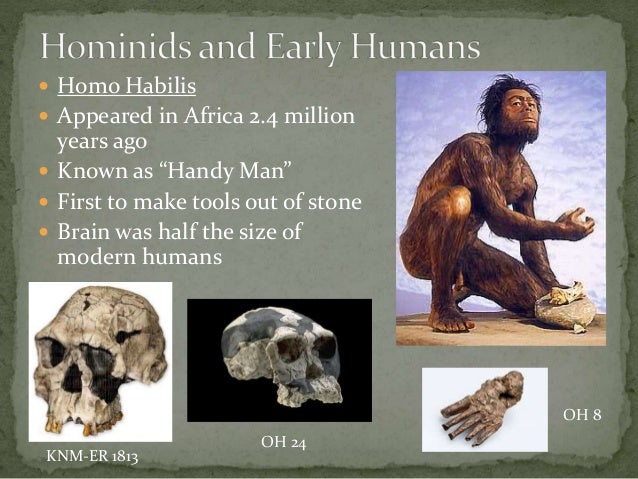This image, which resembles a textbook page or presentation slide about hominids and early humans, features a horizontally aligned layout with a rugged, stone-like background that fades from dark to light gray layers. The main title, "Hominids and Early Humans," is left-aligned at the top in a Times New Roman font with capitalized "H," "E," and "H," and is presented in white text. Below the title, there are yellow bullet points also left-aligned, giving details about Homo habilis: the first bullet point is underlined and states "Homo habilis", followed by additional bullets that provide information: "Appeared in Africa 2.4 million years ago," "Known as 'Handyman'," "First to make tools out of stone," and "Brain was half the size of modern humans."

Beneath these text points, the image includes visual aids: two rectangles containing skull photos—one on a white background labeled "KNM-ER 1813" and the other on a black background labeled "OH24." There is also a smaller rectangle below these, showing what appears to be a fossilized hominid hand labeled "OH8."

In the upper right corner of the image, there is an illustration of a Homo habilis figure. The figure is covered in dark brown hair, with a black goatee and beard but no mustache, short shaggy black hair, and is depicted squatting and looking up to the right. This figure's right arm is bent, holding its palm up loosely, while the left arm is extended to the ground. A white stone object, possibly a tool-in-the-making, is placed before the figure.

Overall, the combination of text and visuals comprehensively details Homo habilis, emphasizing their appearance, geographical origin, tool-making capabilities, and comparative brain size.